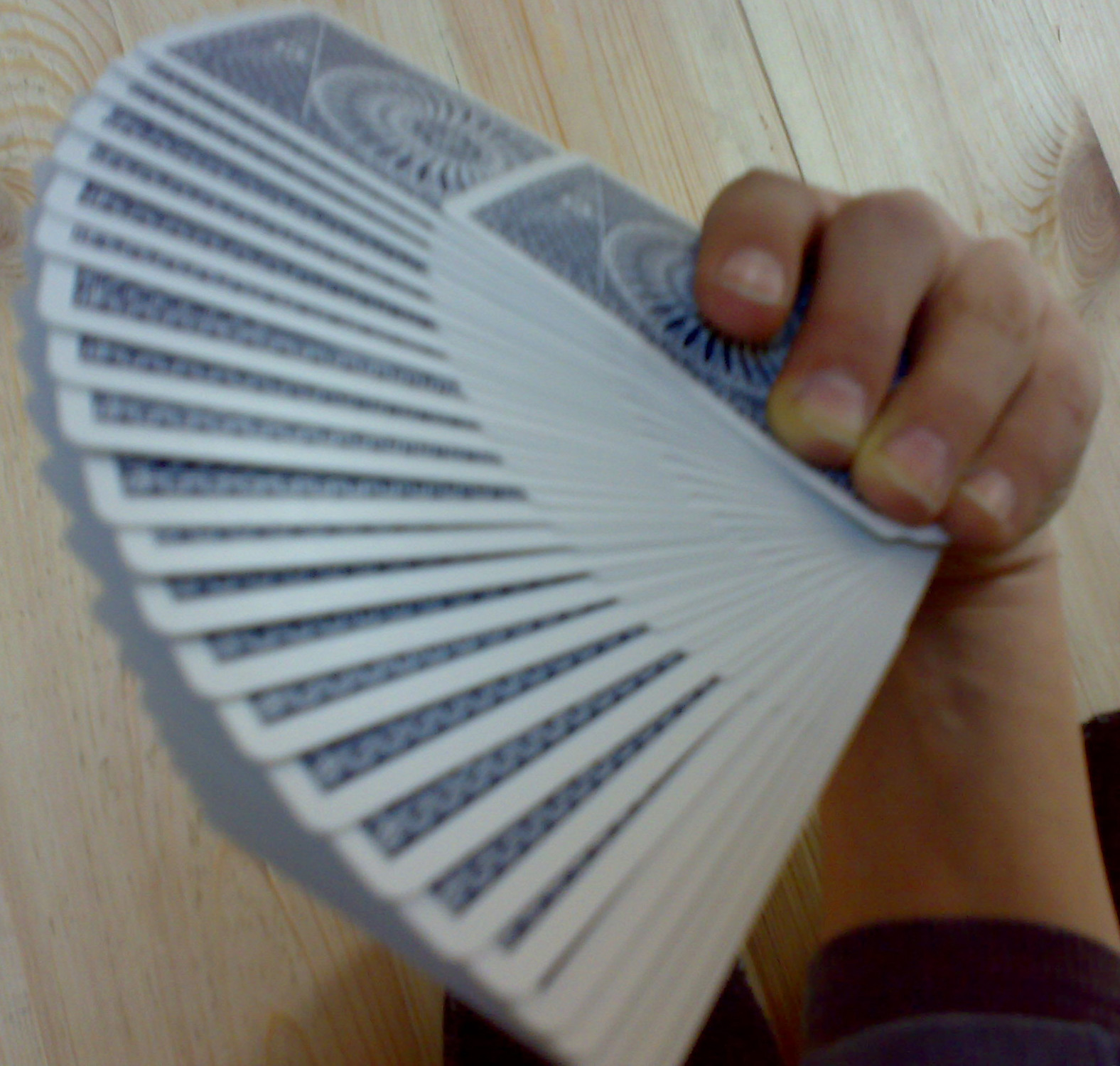The color photograph captures a somewhat blurry, square image of a person holding a fanned-out deck of playing cards. The individual is clad in a long-sleeve black shirt, and their unpainted fingernails are clearly visible. They have skillfully executed a double card fan, with half of the cards fanned near their fingers and the other half extending outward, creating a visually interesting double-decker fan effect. The back of the cards is visible, showcasing a white background adorned with a circular blue pattern at the center. The scene is set against a light-colored wood plank floor, which provides a contrasting backdrop to the darker elements in the image.